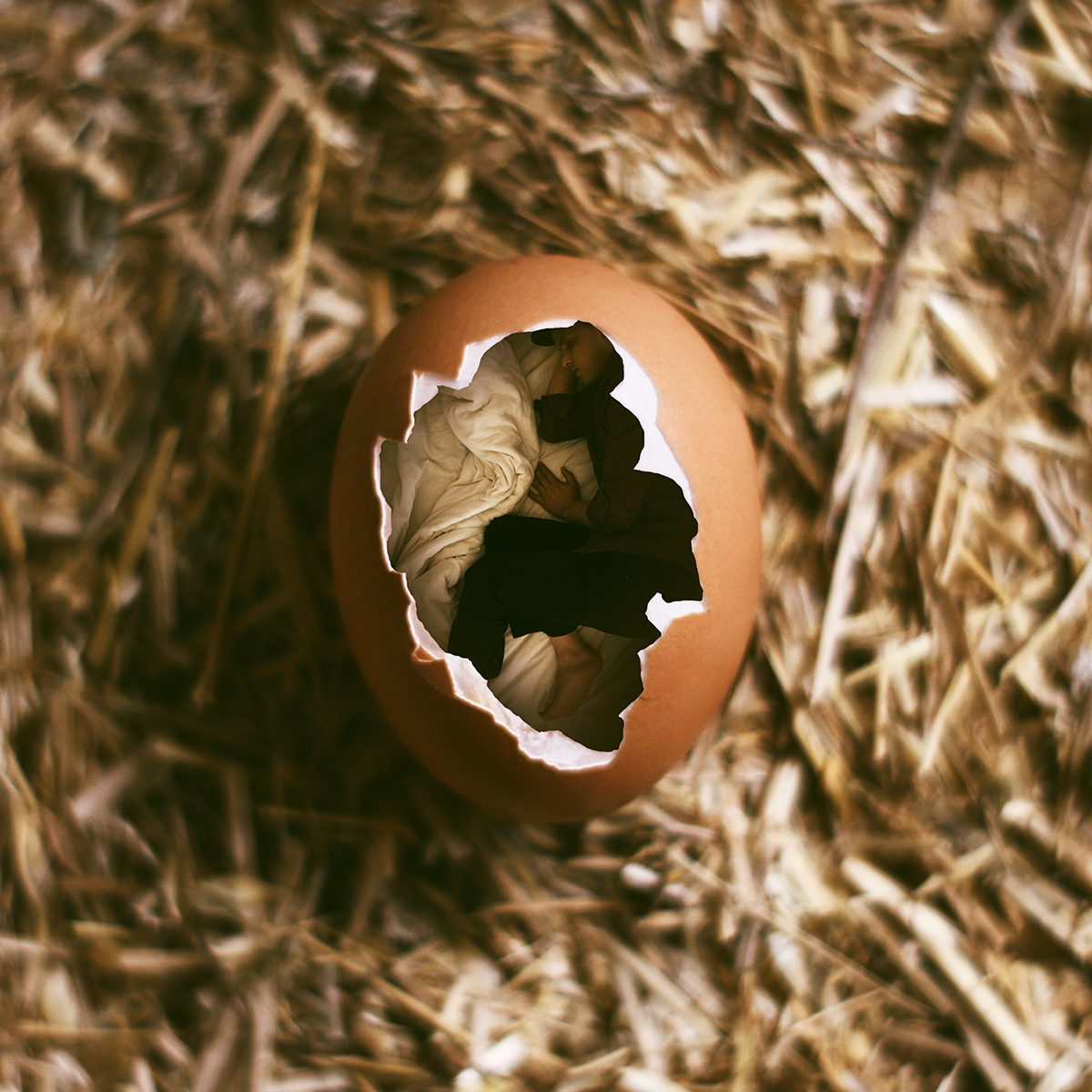The image presents an intriguing optical illusion set against a blurry background of hay or straw. A light-brown egg, cracked open to about 30%, occupies the center of the frame. Inside the egg is not a baby bird, as one might initially think, but a human figure comfortably curled up. This computer-generated or photoshopped illusion reveals the person nestled in white blankets, dressed in black pants and a gray, long-sleeved shirt, and sleeping on their side. The detailed work in creating this illusion is impressive, blending elements of reality with creativity to surprise and intrigue the viewer.